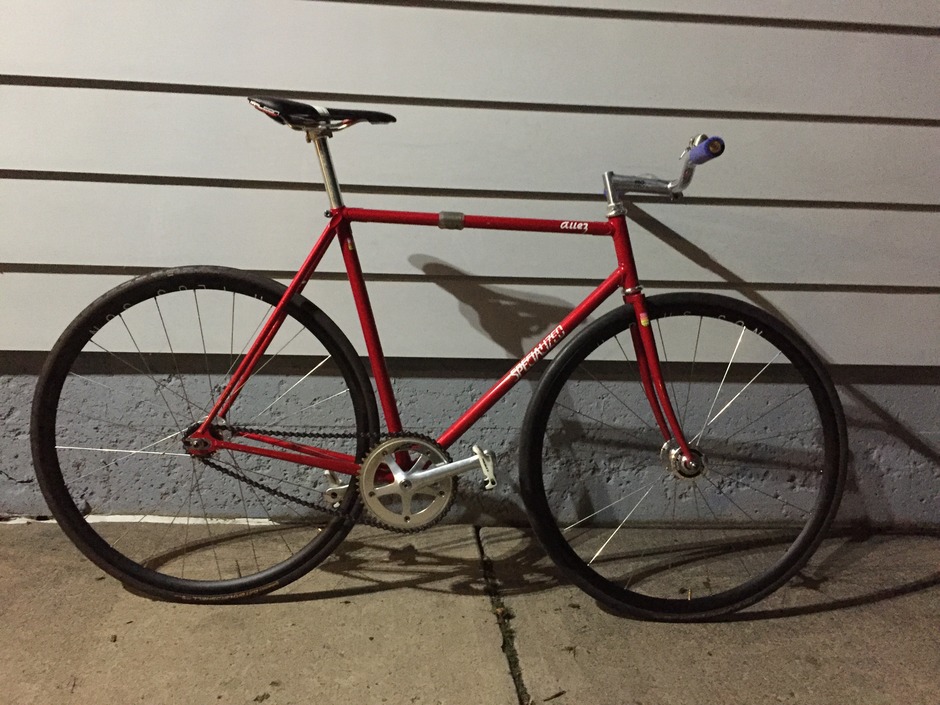This is a detailed photograph of a red-framed bicycle leaning against the side of a light gray house. The bicycle, identified as a Specialized brand, displays the white letters "LA" on the top tube. Its design resembles that of an old racing bike, featuring forward-facing commuter handlebars with a slight dip, rather than the more typical curved racing bars. The handlebars have chrome details and are adorned with a lavender cushion. The bike is equipped with thin, black-rimmed wheels and has a single gear. The seat is a sleek black design with a white stripe. The entire bicycle rests on a standard gray cement driveway, with no kickstand to support it, simply leaning against the house. The house itself is light gray with a foot and a half of block cement foundation visible at the bottom. Areas of the bike, such as the pedals, cranks, and sprocket, are silver, complementing its overall vintage appearance. The photograph emphasizes the solitary presence of the bicycle, highlighting the absence of riders or additional objects.